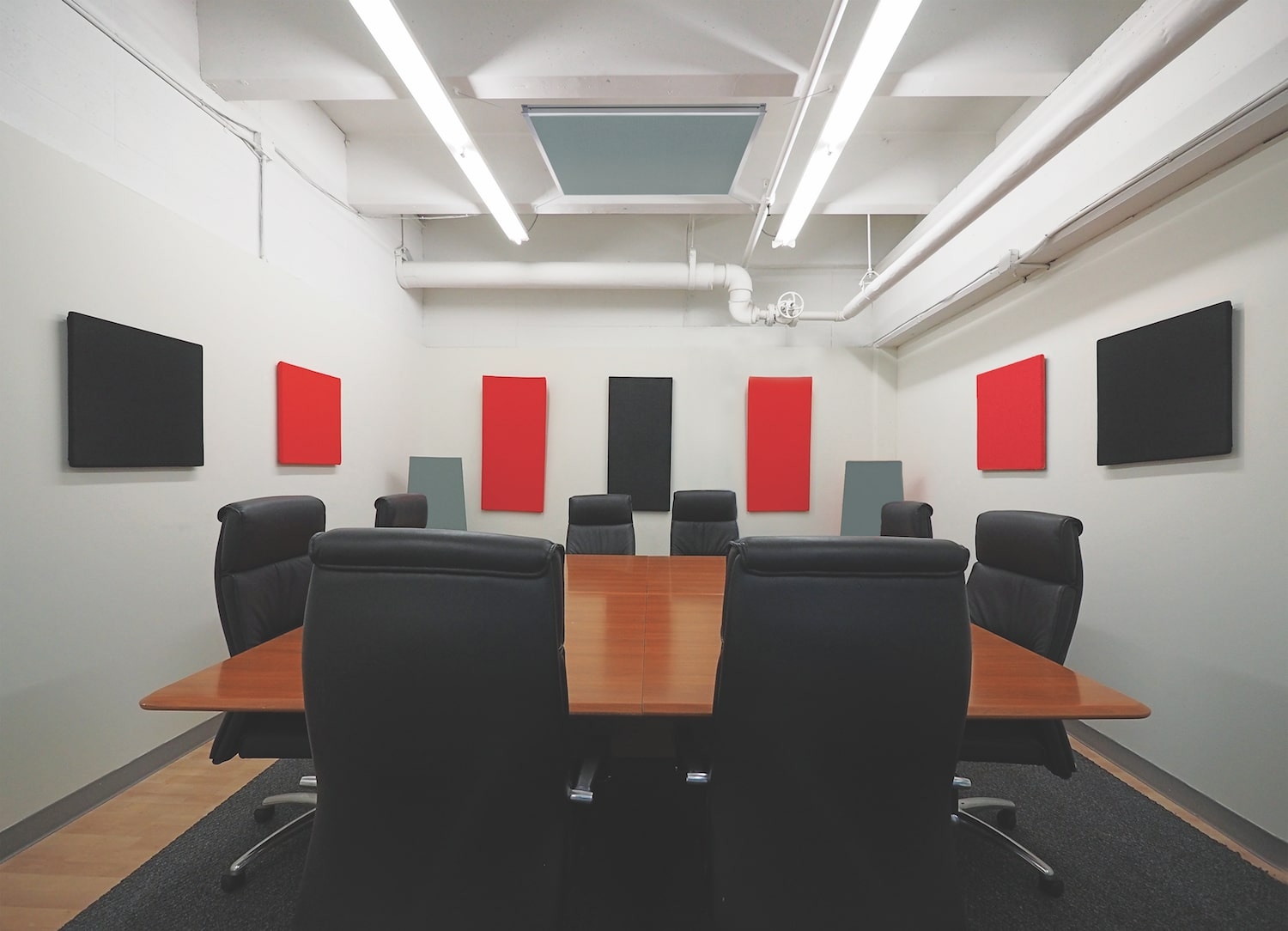The photograph captures a well-lit, industrial-style office space featuring a large, rectangular conference table in the center with a light to medium brown wood top, possibly laminated for a glossy finish. Surrounding the table are eight black, wheeled office chairs, positioned with two on each side. The room is adorned with white or white-gray walls, accented by a gray trim at the bottom. Above, the ceiling showcases exposed pipes and fluorescent lighting, contributing to the room's industrial aesthetic. A large black rug extends under the conference table across the wooden or laminate wood floor. Adding a touch of modern art, the walls display several plain black and red canvas artworks arranged symmetrically. No people are present in this neatly arranged, empty office room.